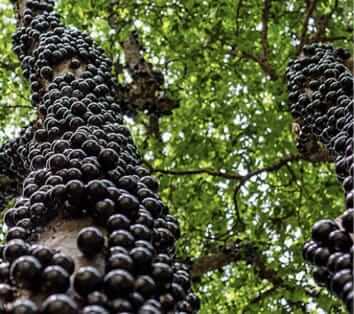This image features the trunks of two tall trees outdoors, both adorned with numerous round, black or brown growths that resemble golf ball-sized plums or small berries. These growths are clustered along the entirety of the visible tree trunks, which makes it intriguing whether they are some kind of fruit, beetles, or disease-induced anomalies like tree galls. The trees, rising prominently in the forest, have branches adorned with green leaves, extending up toward the sky. The background shows daylight filtering through other foliage, emphasizing the natural outdoor setting.